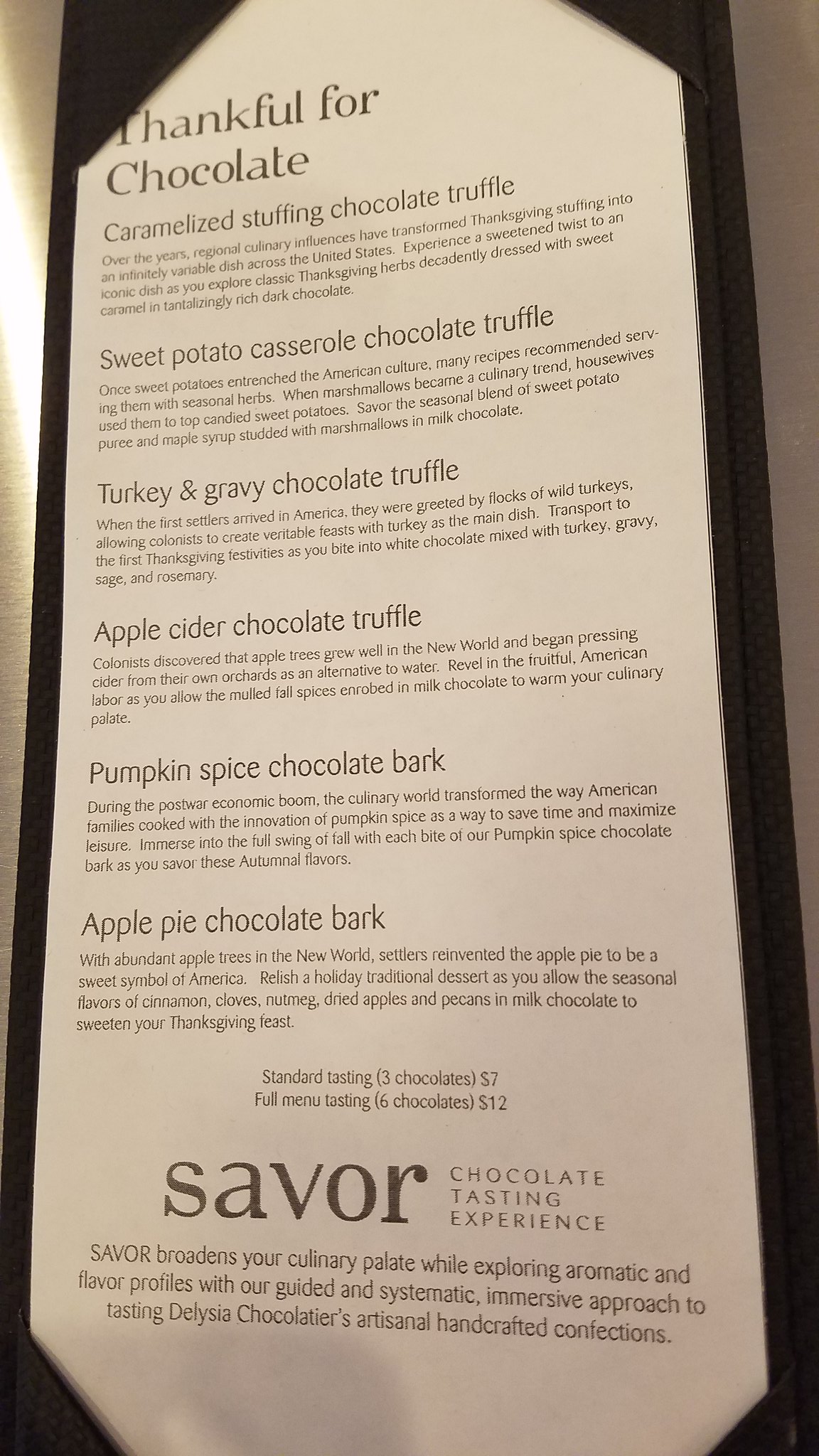This photo showcases a rectangular, black and white menu elegantly presented in a sophisticated black leather slip case. The menu highlights a delectable array of chocolate truffles and barks themed around Thanksgiving flavors. At the top, the menu reads "Thankful for Chocolate."

The first item is a "Caramelized Stuffing Chocolate Truffle," followed by a description in fine print. Next is the "Sweet Potato Casserole Chocolate Truffle," also with an unreadable description due to small font size. This is succeeded by the "Turkey and Gravy Chocolate Truffle," which, like the others, is accompanied by a detailed descriptor. The menu continues with the "Apple Cider Chocolate Truffle," and similarly, a description in small print follows.

The selection then features the "Pumpkin Spice Chocolate Bark," accompanied by a descriptor. Finally, the "Apple Pie Chocolate Bark" appears with another miniature description. Towards the bottom of the menu, pricing is outlined: a standard tasting of three chocolates costs $7, while a full menu tasting of six chocolates is priced at $12.

The menu concludes with the business name, "Savor," prominently displayed in bold font, along with the tagline "chocolate tasting experience." The overall presentation exudes a sense of luxury and culinary adventure.